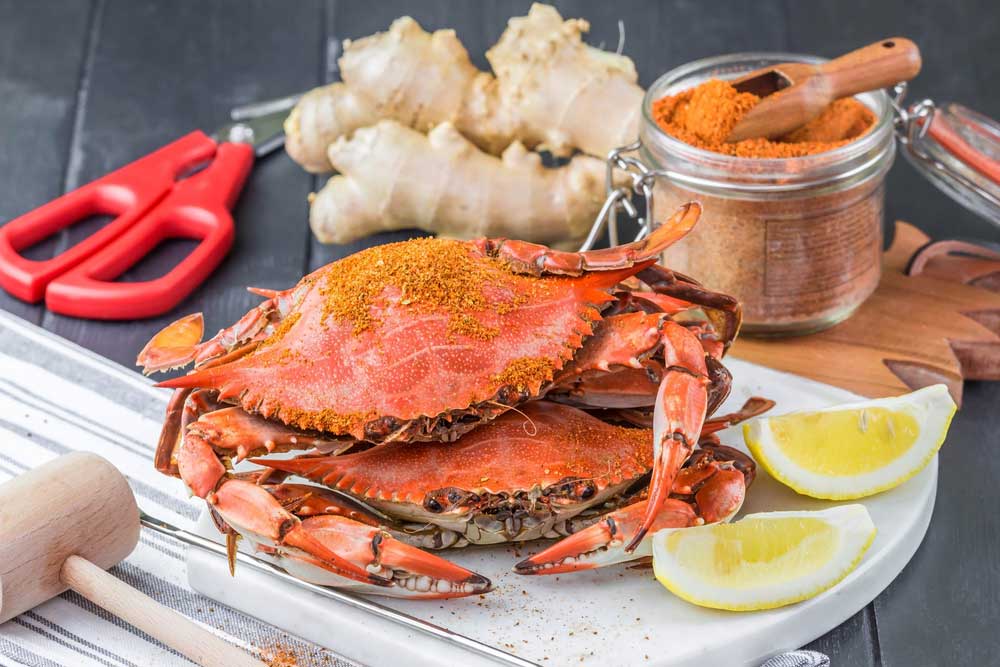This is a detailed image from a prep area of a kitchen, set on a gray multi-slab table or prep area. At the heart of the scene is a white plate on a cutting board, where two burnt orange crabs, still equipped with their claws and shells, are stacked atop each other, dusted with seasoning. To the right of the crabs are two lemon wedges. On the left, a mallet waits, ready to crack open the crabs. Directly behind the crabs, a bowl of orange spices with a wooden spoon invites further flavor, while to the side, a pair of red scissors rests beside what appears to be two large pieces of ginger. The atmosphere suggests preparations for a seafood platter or dinner, meticulously laid out with tools and spices, poised for culinary creation.